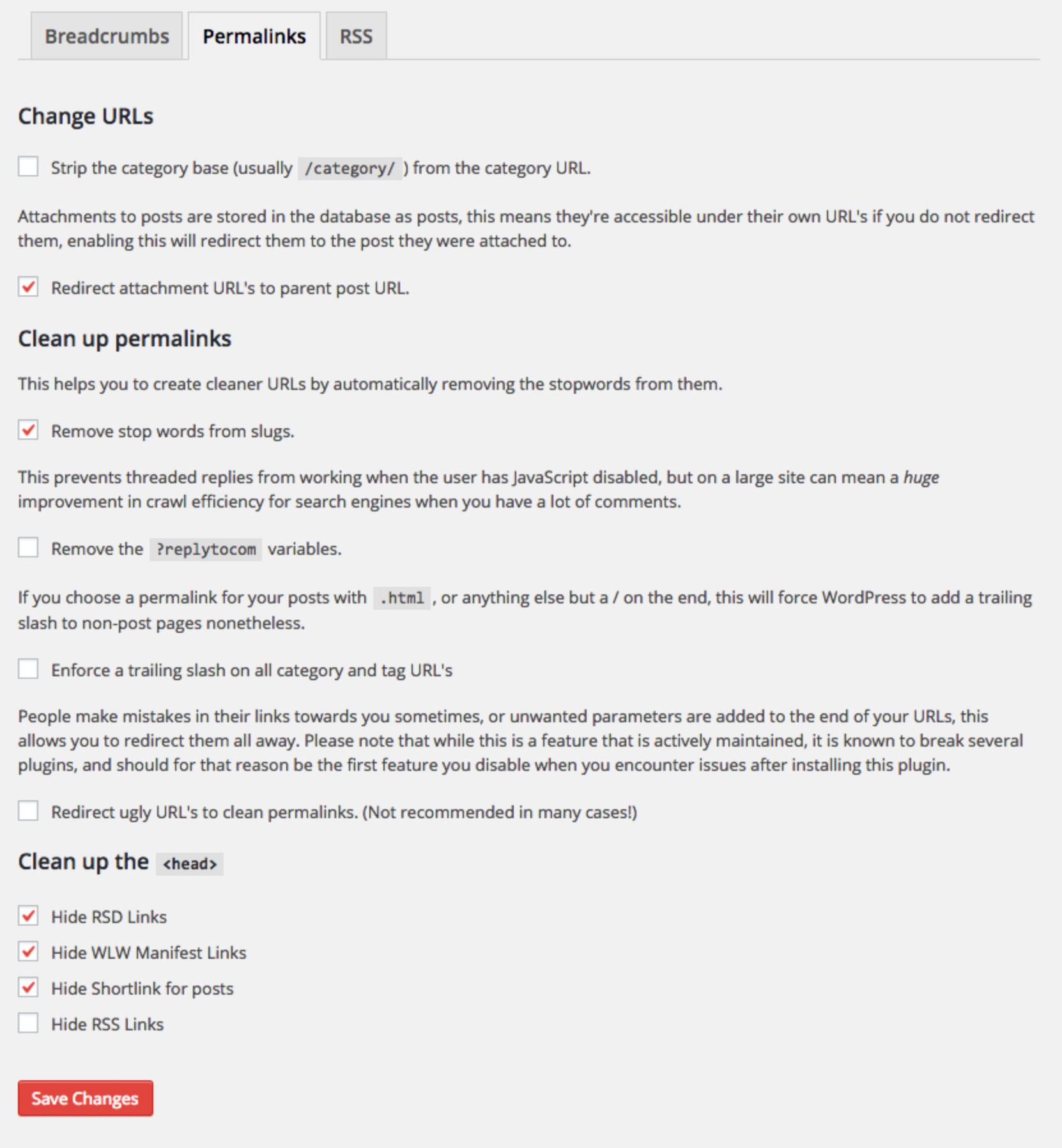In this image, various website configuration and SEO optimization features are displayed. We see categories, breadcrumbs, and amalinks designed for better site navigation and linking. The RSS feed setup is also mentioned. Options for changing URLs are available, including stripping the category base, typically formatted as "forward slash category forward slash," from the category URL for cleaner links. 

Attachments to posts are stored in the database as individual posts, meaning they have their own URLs unless redirected to their parent posts. The option to "Redirect attachment URLs to parent post URL" ensures seamless redirection.

The image also highlights tools like Amalinks Cleaner, which helps create cleaner URLs by automatically removing stop words. The "Remove stop words from slugs" feature further optimizes URL structures.

A specific detail mentions that removing the "reply to com" variables prevents threaded replies from functioning if JavaScript is disabled, but can significantly improve crawl efficiency for search engines on larger sites with many comments.

There's a note on permalink structure preferences, indicating that choosing a format ending with ".html" or other extensions forces WordPress to add a trailing slash to non-post pages regardless.

Overall, the features depicted contribute to a well-optimized, user-friendly website structure.